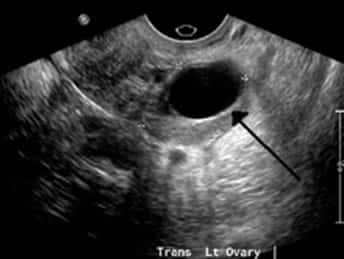This image is a detailed black and white ultrasound of an ovary, labeled "trans LT ovary" at the bottom. The sonogram primarily displays the ovary, indicated by an arrow pointing towards a dark, circular area centrally located within varying shades of gray. The background of the image is mostly black, with some lighter areas that appear as if illuminated by a light. The ultrasound does not show a fetus or any other structures, focusing solely on the ovary. Additionally, at the edge of the image, there is a small, unlabeled scale likely indicating the dimensions of the features being examined. The monochrome nature of the sonogram, typical of such medical imaging, makes it challenging to discern finer details beyond these primary elements.